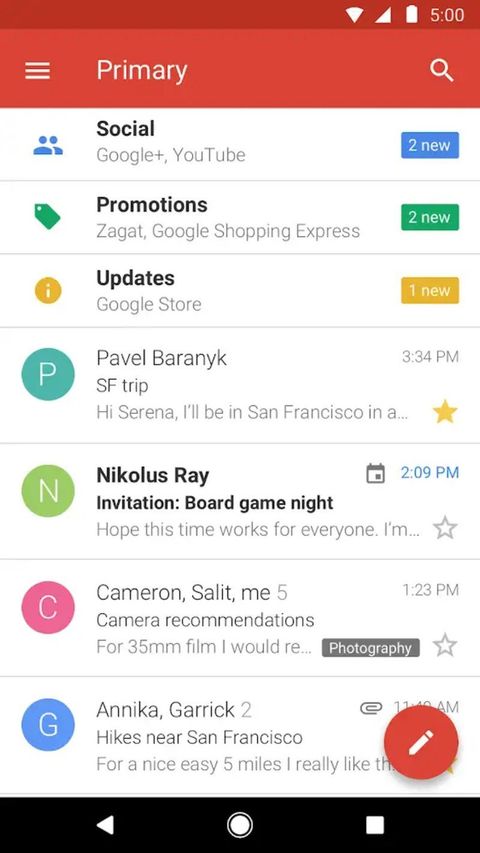This screenshot depicts a mobile phone display showcasing an email inbox at 5:00 PM, indicated by the red bar across the top. The primary folder is selected and features a hamburger menu labeled "Home Primary." The search bar is accessible for quick navigation within the inbox. 

**Primary Folder:**
1. **Social Category:**
   - Google Plus
   - YouTube (2 new items)

2. **Promotions Category:**
   - Zagat
   - Google Shopping Express (2 new items)

3. **Updates Category:**
   - Google Store (1 new update)

4. **Primary Messages:**
   - **Pavel Barnik**: An email about a San Francisco trip, timestamped at 3:34 PM, addressed to "Serena." The message begins with "Hi Serena, I'll be in San Francisco in a..." and includes a star, signifying importance.
   - **Nicholas Ray**: An unread email regarding an "Invitation for Board Game Night," mentioning a proposed time and seeking confirmation from recipients.
   - **Cameron Sollet**: A discussion thread including the user and Cameron Sollet, featuring recommendations on camera choices.

The visual representation highlights the various categories and their corresponding notifications, providing a snapshot of the user's email activities and pending messages requiring their attention.